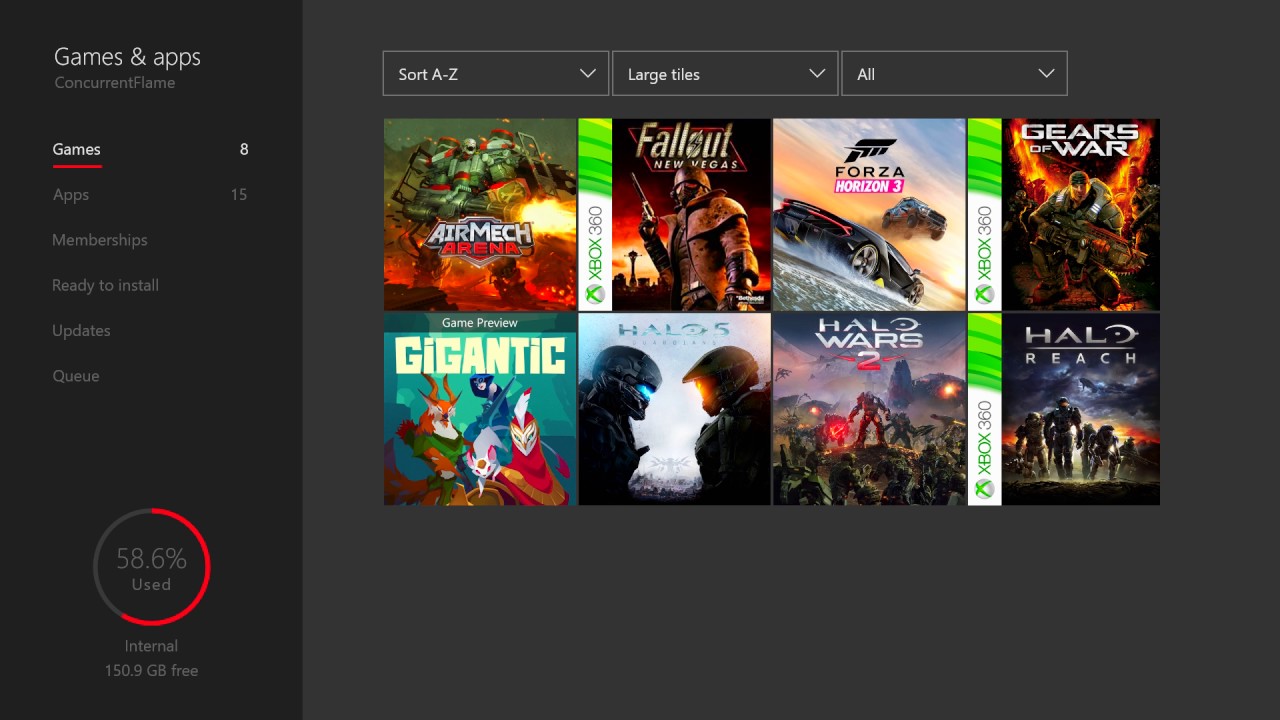This screenshot, likely taken from a laptop, showcases a detailed interface view of a gaming and app management system. On the upper section, two distinct columns are visible. The left-hand column, set against a black background, is headed by the titles "Games & Apps" and "Concurrent Flame." Below this, the section "Games" is highlighted with a red underline, displaying a count of 8, followed by "Apps" showing a count of 15. Further down, subsections titled "Memberships," "Ready to Install," "Updates," and "Queue" are listed. At the bottom of this column, a storage usage indicator reads "58.6% Used" within a red-highlighted circle, with a note stating "Internal: 150.9 GB Free."

In the main area of the screenshot, there are three buttons labeled "Sort A-Z," "Large Tiles," and "All." The content area is divided into a grid format, presenting four tiles across two rows. The visible tiles include:
1. "AirMech Arena"
2. "Fallout: New Vegas"
3. "Forza Horizon 3"
4. "Gears of War"
5. "Game Preview Gigantic"
6. "Halo Wars 2"
7. "Halo Reach"

This user's screenshot appears to offer a comprehensive overview of available gaming options, perhaps shared to facilitate deciding what game to play next or to arrange co-op gameplay sessions with friends, as these games typically require significant time investment.